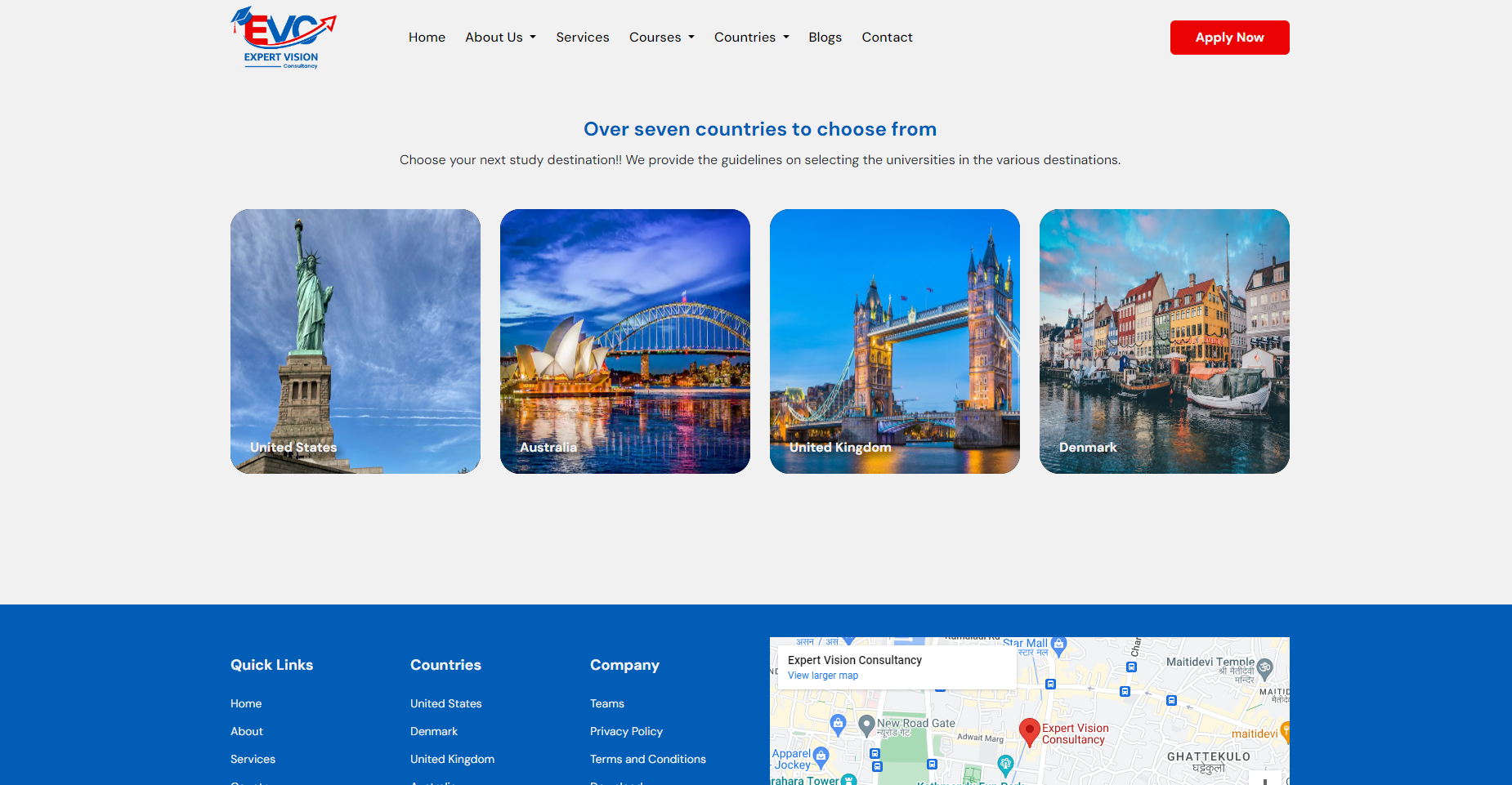The image is a screenshot from a website labeled EBC. The webpage background is a light gray color. In the upper left corner, there is a logo featuring arrows swirling around the letters "EBC." The "E" is a capital letter in red, while both the "V" and "C" are capital letters in blue. Below the logo, there is accompanying text.

At the top center of the image, there are several navigation tabs labeled "Home," "About Us," "Services," "Courses," "Blogs," and "Contact." In the top right corner, there is a prominent red "Apply Now" button.

The central part of the image features a headline stating "Over Seven Countries to Choose From," and more detailed information is provided below this statement. Beneath this section, there are four images representing different locations: Denmark, the United Kingdom, the United States, and an indiscernible fourth location. At the bottom of the image, there is a map for additional context.